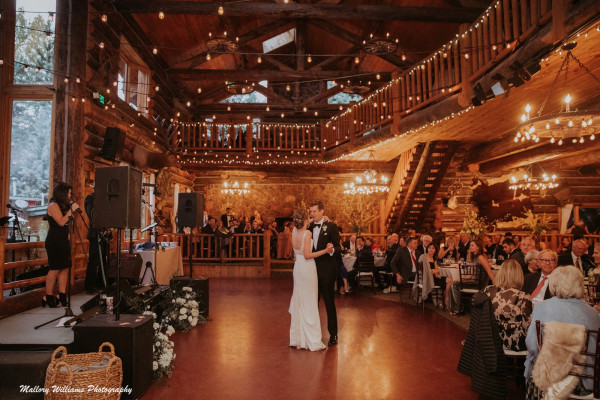The photograph captures a picturesque winter wedding set in a grand, two-story log cabin, possibly within a ski resort, as suggested by the visible snow outside. The scene is intimate yet expansive, with exposed wood rafters and floor-to-ceiling rectangular windows framing the interior. At the center of the image, the bride, in a white strappy gown, shares a tender dance with the groom on a spacious, empty dance floor. Guests, elegantly dressed in suits and gowns, are seated at tables around the dance floor, attentively watching the couple.

To the left, a small stage adorned with white flowers hosts a woman in a black dress, likely performing a song. Black cube speakers frame the stage, adding to the cozy yet sophisticated ambiance. Above, a loft-type balcony is strung with delicate white Christmas lights, enhancing the romantic atmosphere. The image, in a rectangular format with its long sides at the top and bottom, features the watermark "Mallory Williams Photography" in cursive at the bottom left corner.